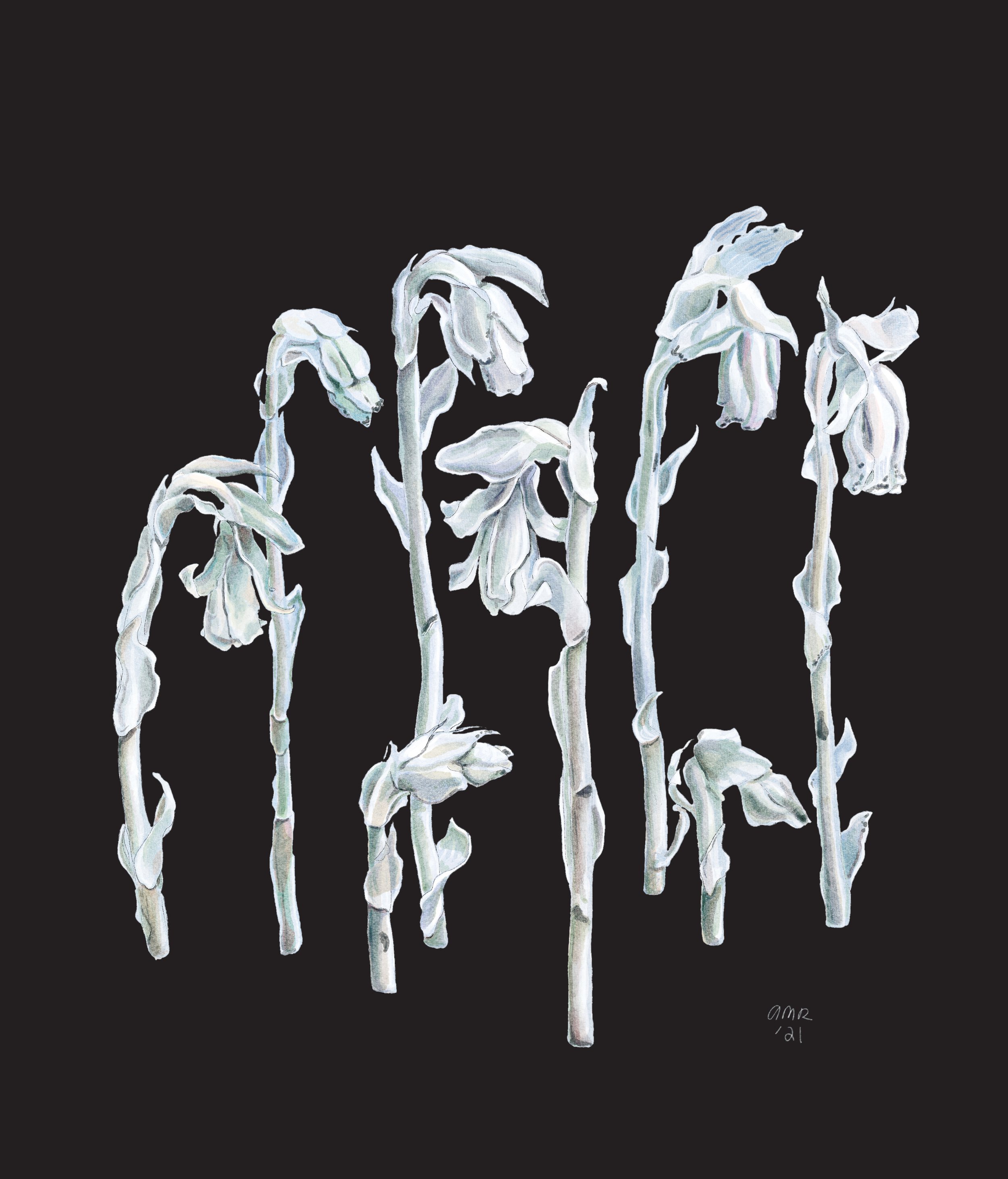This detailed painting, possibly digital, titled "AMR 21" in the bottom right corner, features a striking depiction of eight Indian Pipe flowers against a rich, velvet-like black background. The stalks, painted in delicate shades of grayish-white, exhibit a haunting beauty reminiscent of frozen or dead white flowers. Most notably, the flowers' heads droop downward as if wilting, conveying a somber yet captivating elegance. The image includes six larger, taller stalks along with two shorter ones, all adorned with leaves pressed against their stalks but not yet unfurled. One central stalk stands prominently closer to the viewer, drawing the gaze forward while the rest recede into the background, enhancing the depth and composition of this evocative art piece.